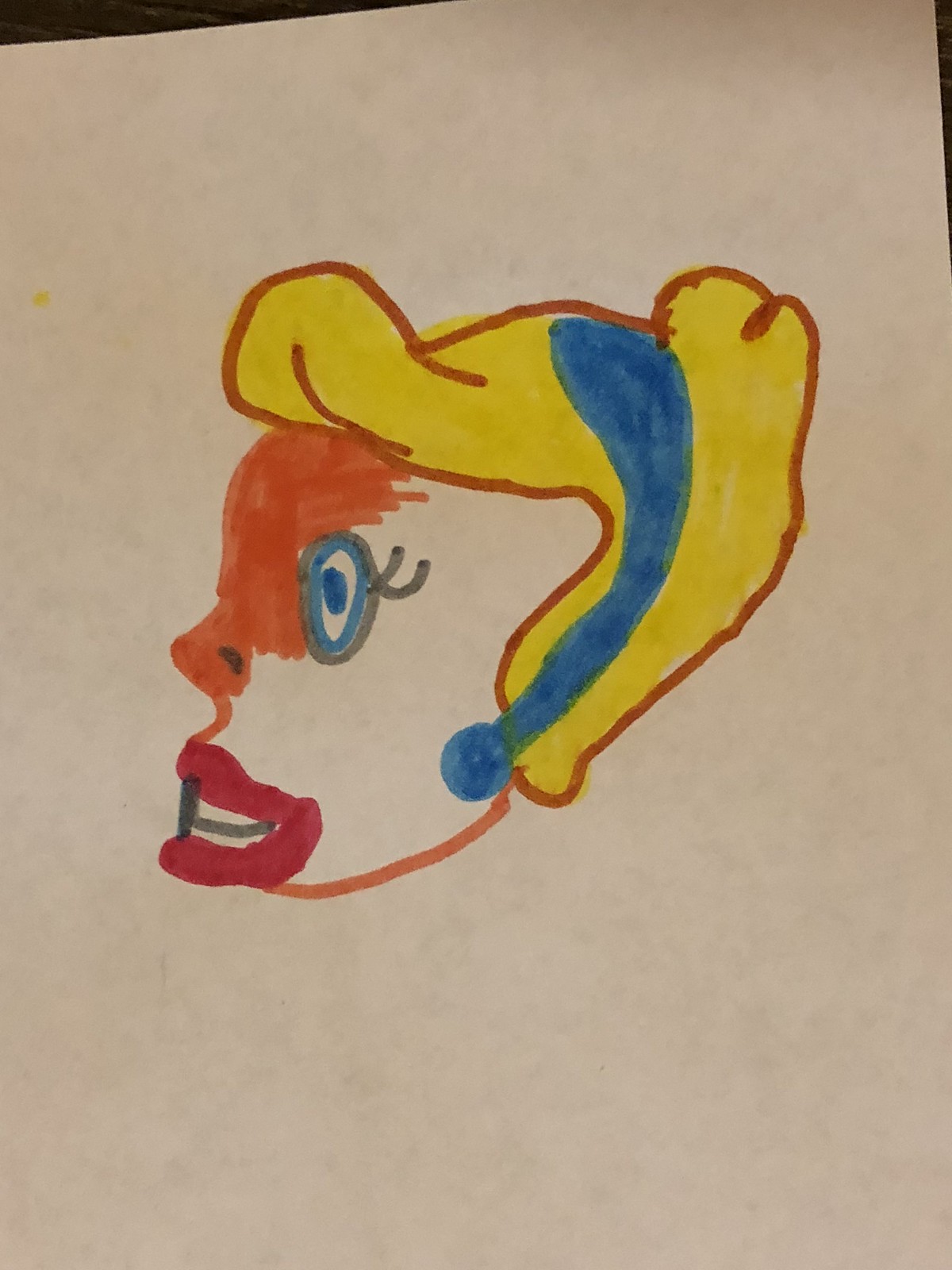This image features a partially colored cartoon-style side profile of a woman's face, likely sketched with markers. The artwork is on a tan-colored paper, framed by a brown outer border. The woman has bright yellow hair that swoops back from her forehead and cascades downward. She wears a blue headband, which might be a ribbon or bow, stretching from ear to ear over the top of her head and ending in a blue dot near her ear.

Her eyes are blue with two distinct black eyelashes extending from the side. The face, predominantly white, shows hints of medium brown coloring around the nose and upper forehead. The nose includes a small black nostril. The lips, painted a deep red, part to expose two rows of teeth separated by a gray line.

Although the drawing appears unfinished, with some areas of the face merely outlined in orange and peach hues, it exudes a whimsical charm reminiscent of Cinderella due to the blonde hair and the iconic blue headband. The attention to detail suggests a youthful artist at work, blending simple lines with vivid colors.